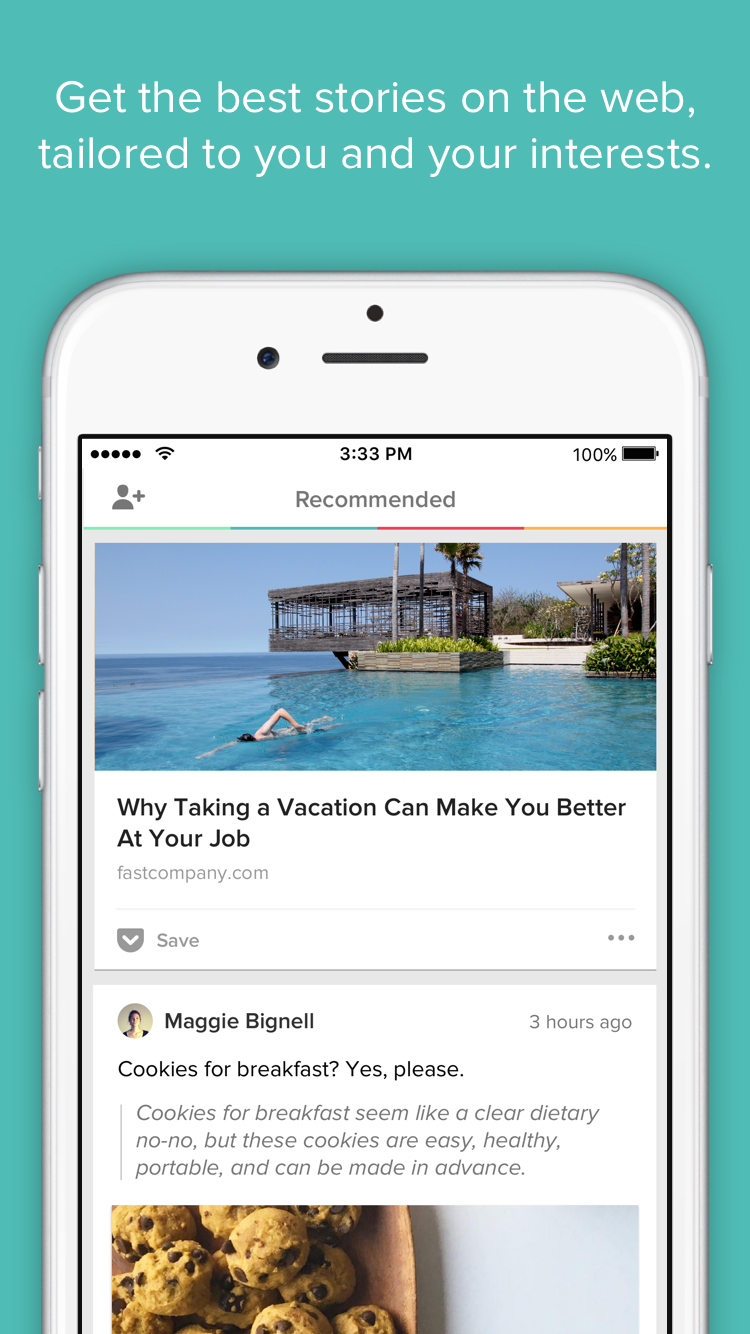**Caption:**

A visually appealing advertisement is set against a striking turquoise blue background. At the top, in crisp white lettering, reads the tagline: "Get the best stories on the web, tailored to you and your interest." Below this, a gray-outlined smartphone is prominently displayed with a white screen. 

The top section of the phone screen features a typical smartphone status bar: on the left, five dark circles indicating Wi-Fi signal strength and an icon of a person with a plus sign; on the right, a battery icon filled in black at 100%, along with the time "3:33 p.m." in black text. Just below, the word "Recommended" appears in black on the same white background. 

A vibrant, multicolored banner spans the top, transitioning from greenish-blue to blue, red, and yellow. This banner introduces a captivating image beneath it: a breathtaking snapshot of a person swimming in the ocean against the backdrop of a picturesque scene, reminiscent of destinations like Bali, Malaysia, or the Philippines.

Highlighted beneath this image is an article title in black text: "Why taking a vacation may make you better at your job" by Fast Company. Below, another story by Maggie Bignell is shown, featuring her icon beside her name. The title reads, "Cookies for breakfast? Yes, please." It entices with a promise of easy and healthy breakfast cookies. Accompanying this is an inviting image of a brown plate stacked with what appear to be delicious chocolate chip cookies.